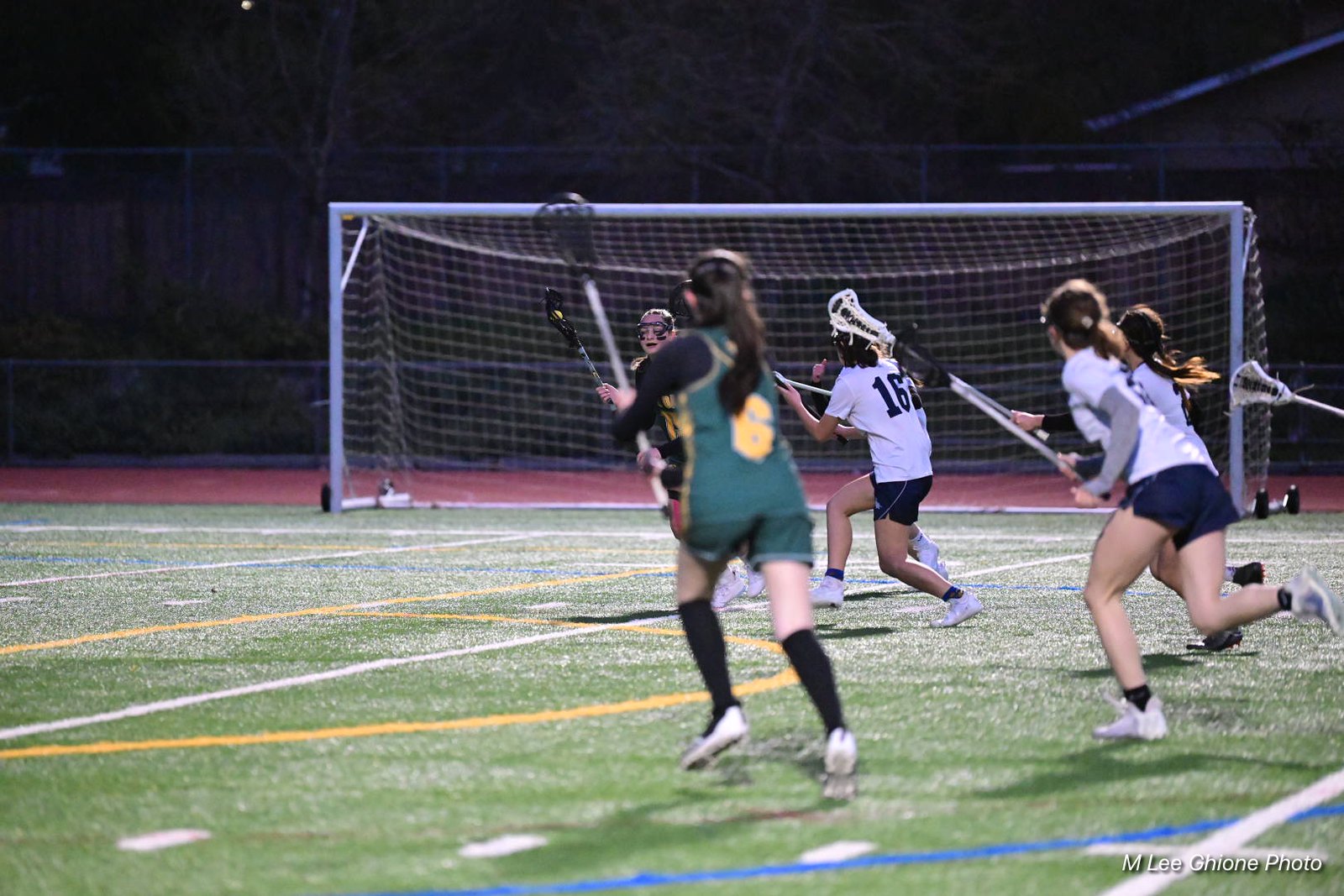The photograph captures a nighttime field lacrosse game, set on a meticulously maintained artificial green field marked with yellow, white, and blue lines. The scene centers on five female players in action, racing toward a large white goal with a net situated against a black sky backdrop. Behind the goal is a red track field, encircled by a series of chain-link and wooden fences, and the faintly visible tops of houses.

On the offensive side, three girls clad in white jerseys with black pants and socks are seen rushing the goal. Closest to the camera, a girl in a green jersey and shorts, marked by a yellow symbol on her back, is prominently visible holding a lacrosse stick. Opposite these attackers, partially obscured by the girl in green, stands the goalie in darker attire, positioned to guard the net. Another player in green can be seen on the mid right side of the image, with her lacrosse stick extending into the frame. The red track field in the background suggests the full extent of the playing field, subtly hinting at the broader scale of the sports complex.